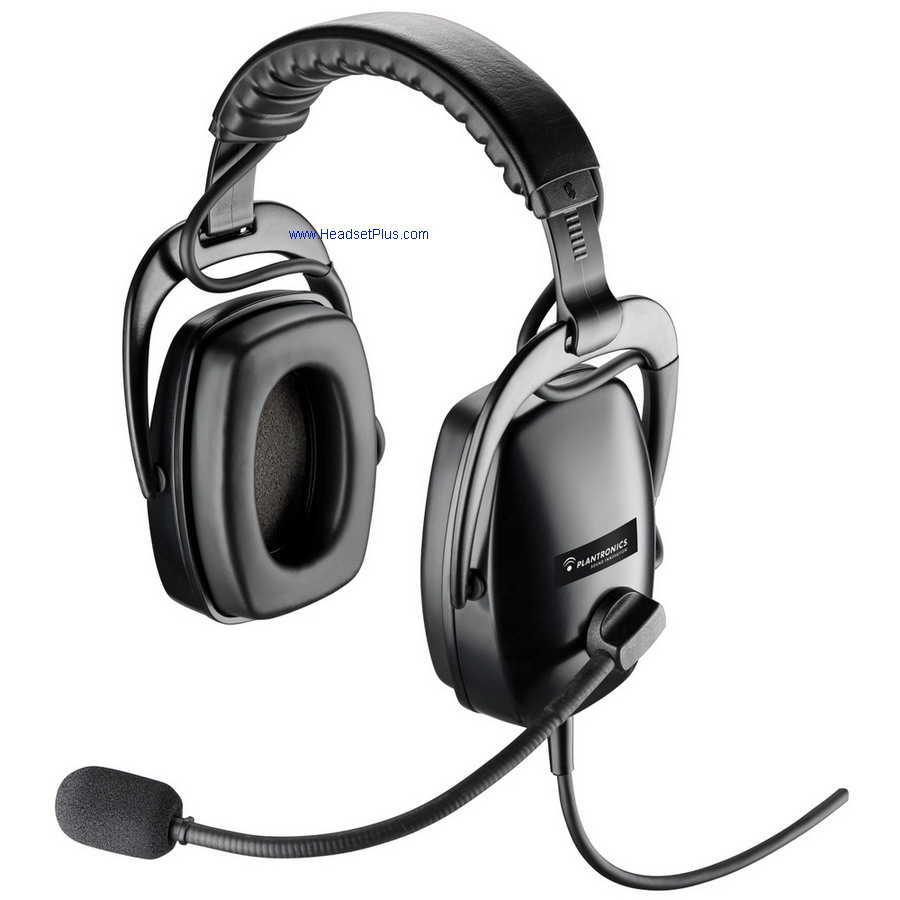This is a detailed photograph of a high-quality gaming headset, predominantly black in color, set against a clean, white background. The headset features large, square foam earmuffs that cover the ears completely for an immersive audio experience, as well as a cushioned band that sits comfortably over the top of the head. A black, movable microphone with a grayish fuzzy tip extends from one of the earmuffs, enhancing the communication capability of the device. Additionally, a black wire descends from the left earpiece. Towards the upper left corner of the image, there's a small blueprint with the URL "www.headsetplus.com" in blue, indicating the likely source or retailer of the headset. Overall, the image presents the headset in a clear and detailed manner, highlighting its design and features, suggesting it is well-suited for gaming and other communicative activities.